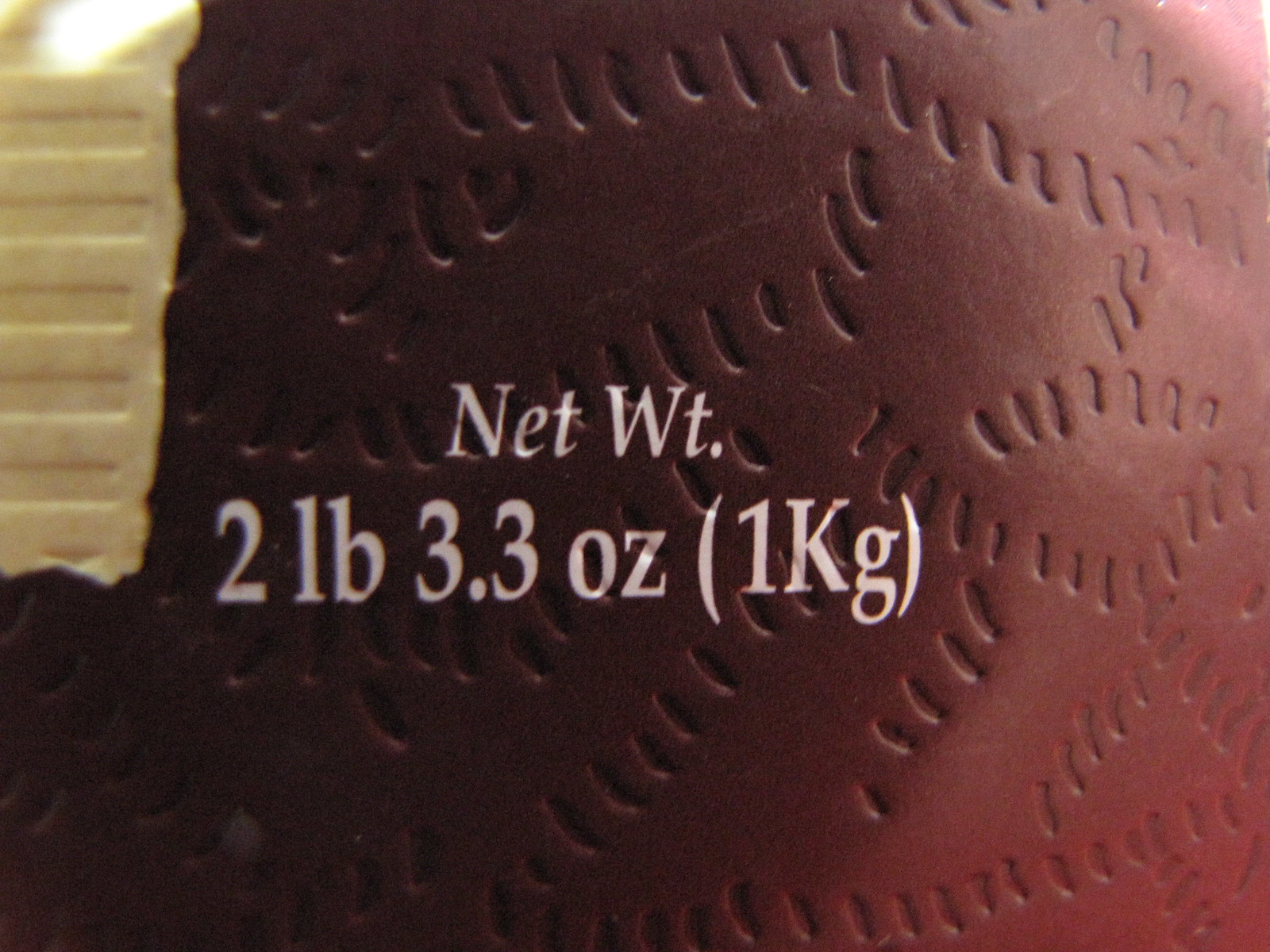This photograph features a red object with indentations that closely resemble the stitches of a baseball, although the object itself is not a ball. In the upper left-hand corner, part of a white plastic shelf is visible. The shelf has text printed on it, which includes the following weight measurements: "NET WT." (abbreviation for Net Weight), followed by "2 LB" (2 pounds), "3.30 OZ" (ounces), and "1 Kg" (1 kilogram). The exact nature or purpose of the red object remains unidentified, but the detailed labeling provides clear information about its weight.